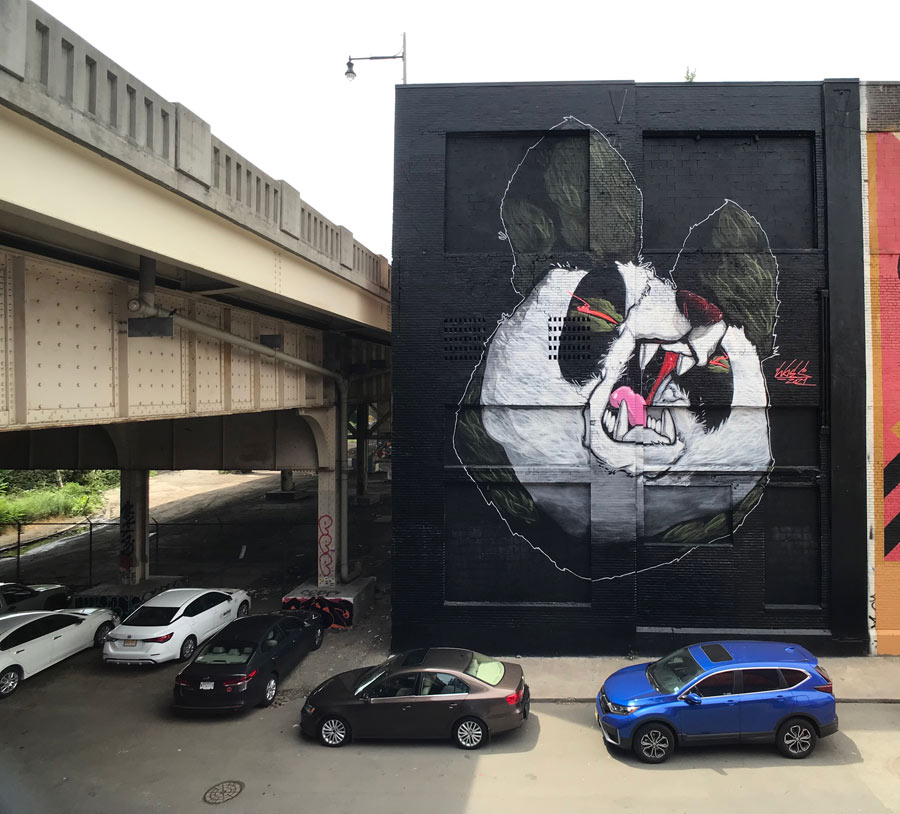This square, outdoor photograph, six inches by six inches, captures a striking urban scene during the daytime. Dominating the composition is a large, black-painted, three-story brick building with no windows on its visible side, possibly an industrial structure. The central feature of the image is an immense graffiti mural of an aggressive animal's head—likely a panda, though with exceptionally large, almost mouse-like ears that add an intriguing twist to its appearance. The mural's face is primarily white, contrasted by dark, almost greenish-black fur around its angry red eyes, and black ears. The open mouth reveals sharp, fanged teeth and a pink tongue, contributing to its menacing expression. The mural is also tagged with red paint on the right side. Below the building is a street with a sidewalk, where several cars, including a blue SUV and a gray sedan, are parked. To the left, a concrete highway overpass extends from the upper left corner, with visible girders and steel slats underneath, reaching towards the lower center of the photo. Cars are parked beneath the overpass and on the street in front of the building, with greenery and a sidewalk partially visible in the left center.